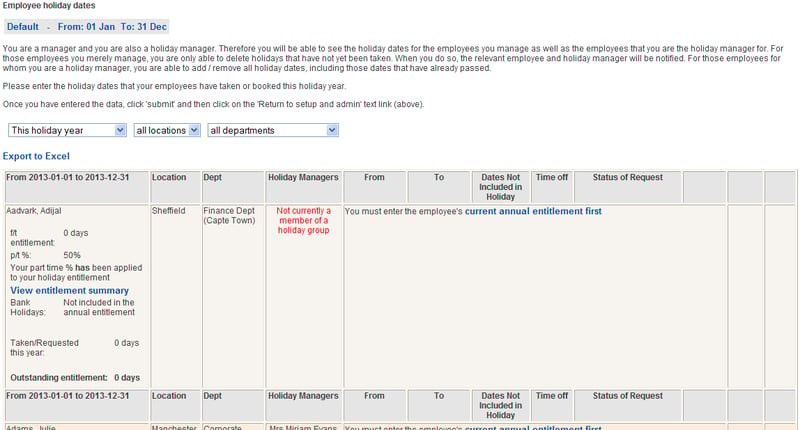**Caption:**

This screen capture displays an employee holiday management and tracking system interface. In the upper left corner, there is a header titled "Employee Holiday Dates," which spans the default period from January to December. An informational blurb below the header explains user roles and visibility permissions: as both a manager and a holiday manager, you can view holiday dates for the employees you manage, as well as those you oversee as a holiday manager. For employees you only manage, you can see and delete holidays that have been used or taken, and upon doing so, relevant employees and holiday managers will be notified. However, as a holiday manager, you have the authority to add, remove, and modify all holiday dates, including past dates. 

The interface includes a feature labeled "Export to Excel," providing the ability to export data. Below this, a detailed grid or form is displayed, outlining critical information such as the date of the holidays, location, department, holiday manager, duration (from-to), dates not included in holidays, time off, and status. The matrix at the bottom offers a comprehensive view: the left side lists who is entitled to employee dates, while the right side details pertinent information like the location and department.